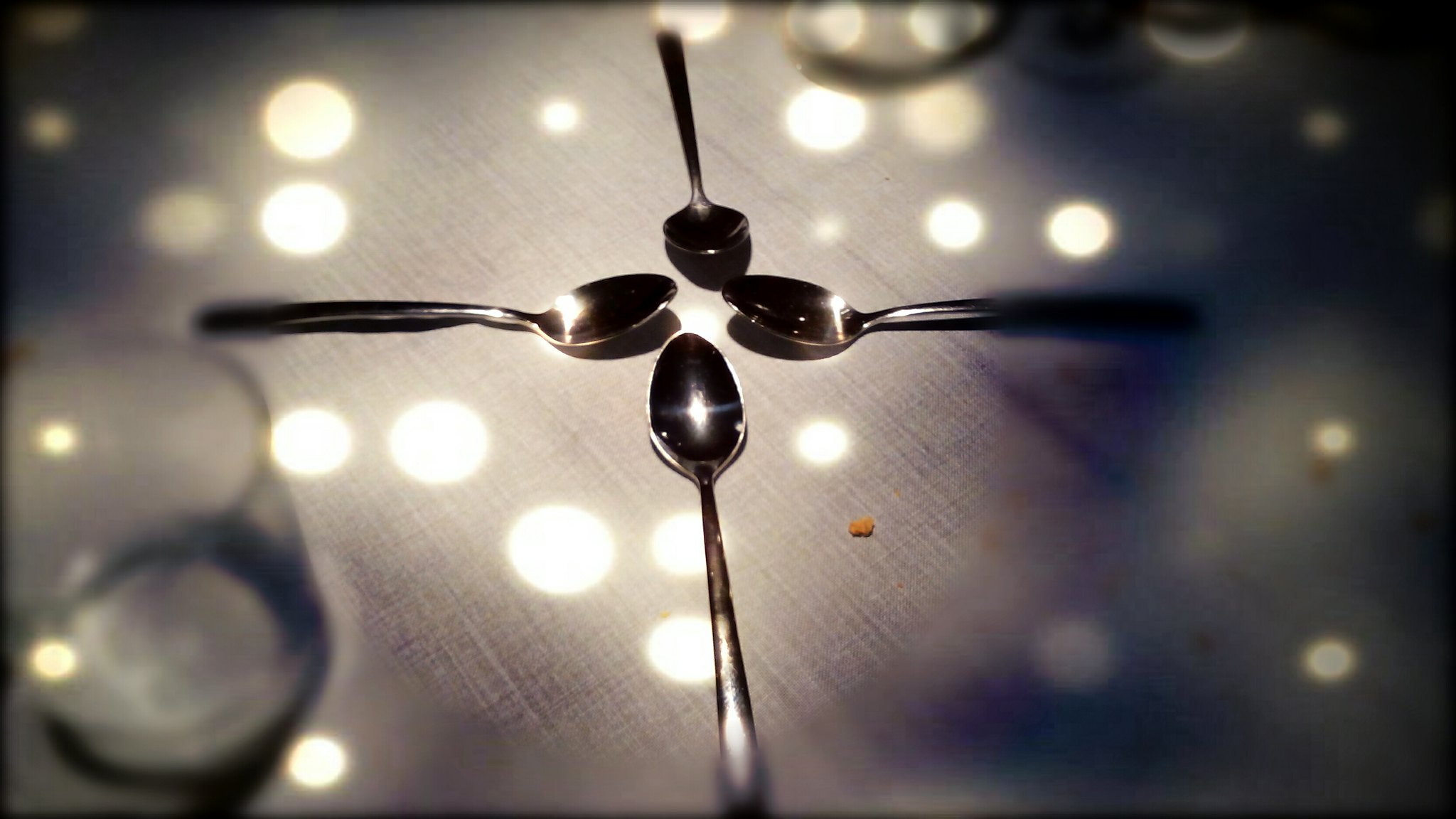In this image, four metallic spoons are arranged with their heads pointing towards each other, forming a square-like pattern. Positioned on a gray, linen-like tablecloth, the spoons reflect light from above, creating bright white dots scattered across the image. Among these dots, around twenty varying in brightness, there is a noticeable crumb situated between two of the spoons. The gray background is somewhat ambiguous, suggesting either a table or a cloth. To the left and upper parts of the image, out-of-focus clear glass cups can be seen, adding depth but remaining secondary to the sharply focused spoons in the center. The overall design is unmarked by text, leaving its purpose and the origin of the light dots a mystery.